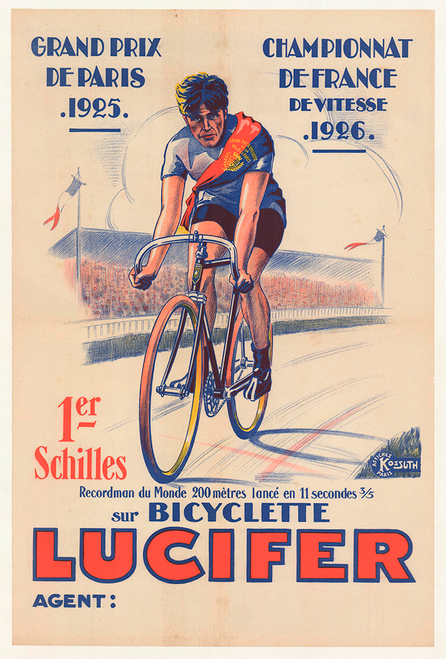The light pink poster showcases a vibrant colored drawing of a man riding a bicycle, wearing a blue shirt with an orange sash extending from his right shoulder to his left side, and black shorts. He grips the uniquely designed handlebars at the bottom ends. The bicycle's front tire is colored with orange on top and yellow at the bottom, appearing translucent without visible spokes. The background depicts crowds, suggesting a lively event atmosphere. The text details include "Grand Prix de Paris 1925" in the upper left corner and "Championnat de France de Vitesse 1926" in the upper right. Below the cyclist, it reads "1ER Schilles" followed by "Recordement de Monde 200m L'Anse in 11 seconds 3/5 sur Bicyclette." Near the bottom in red, outlined in blue, it says "Lucifer," and beneath that, "Agent Cohen."